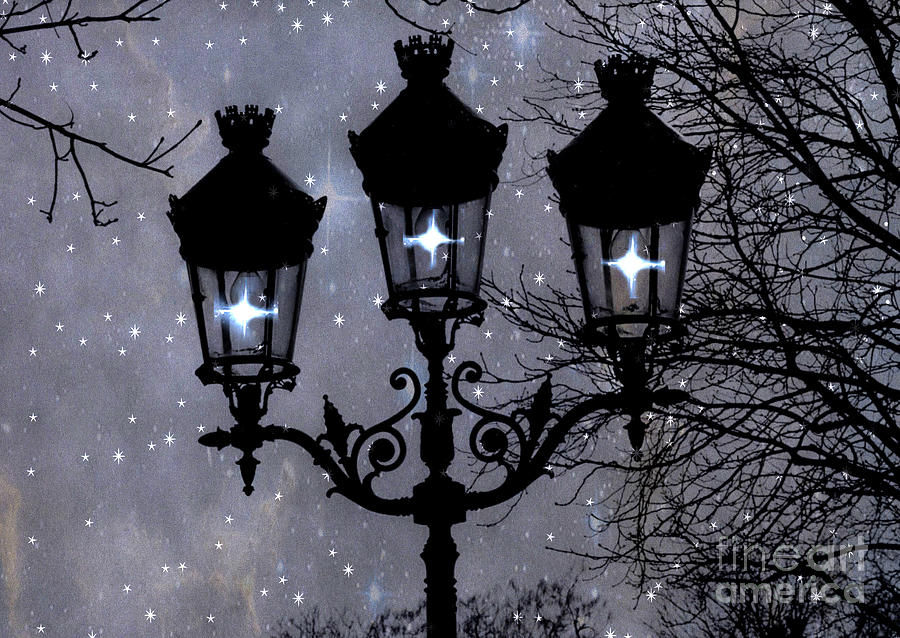In the foreground of this artistic depiction, a tall, intricate black lamppost stands prominently, resembling the gas lights from 1800s Paris. Mounted atop the lamppost are three spherical lights, encased in glass and emitting a bright white and blue glow. The lamppost has a small crown-like detail at its peak, contributing to its vintage charm. Bare black tree branches extend from both sides of the image, adding a stark contrast to the brightly illuminated lamps. The background portrays a snowy night with a vivid, gradient sky filled with artificial white stars and swirling galaxy colors in blues, yellows, and oranges. The scene is markedly detailed with deep blacks and bright whites, enhancing the image's dramatic contrast. In the bottom right corner, there is a watermark that reads "Fine Art America."